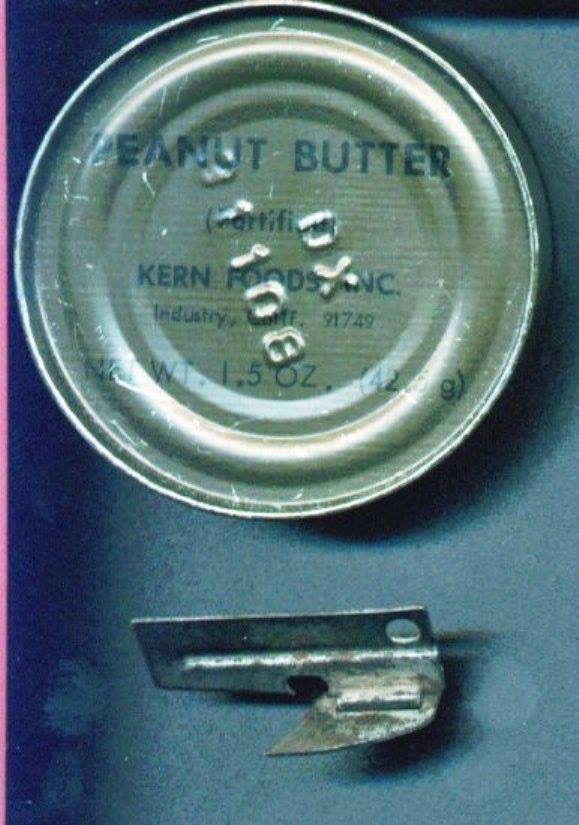The image captures a vintage tin of peanut butter with a brass lid engraved with the codes "A1108" and "DX." The lid features a concentric circular pattern and prominently displays the text "Peanut Butter Fortified" followed by "Kern Foods Inc." in blue lettering. Additionally, it includes the inscription "Industry 91749" and indicates a net weight of "1.5 ounces, 42 grams." The tin is positioned against a teal blue surface. Below the tin, there is a rusted, small handheld can opener with a fold-out blade and a small rectangle with holes, typically used for camping. The background gives a worn, grayish tone, adding to the vintage feel of the scene.